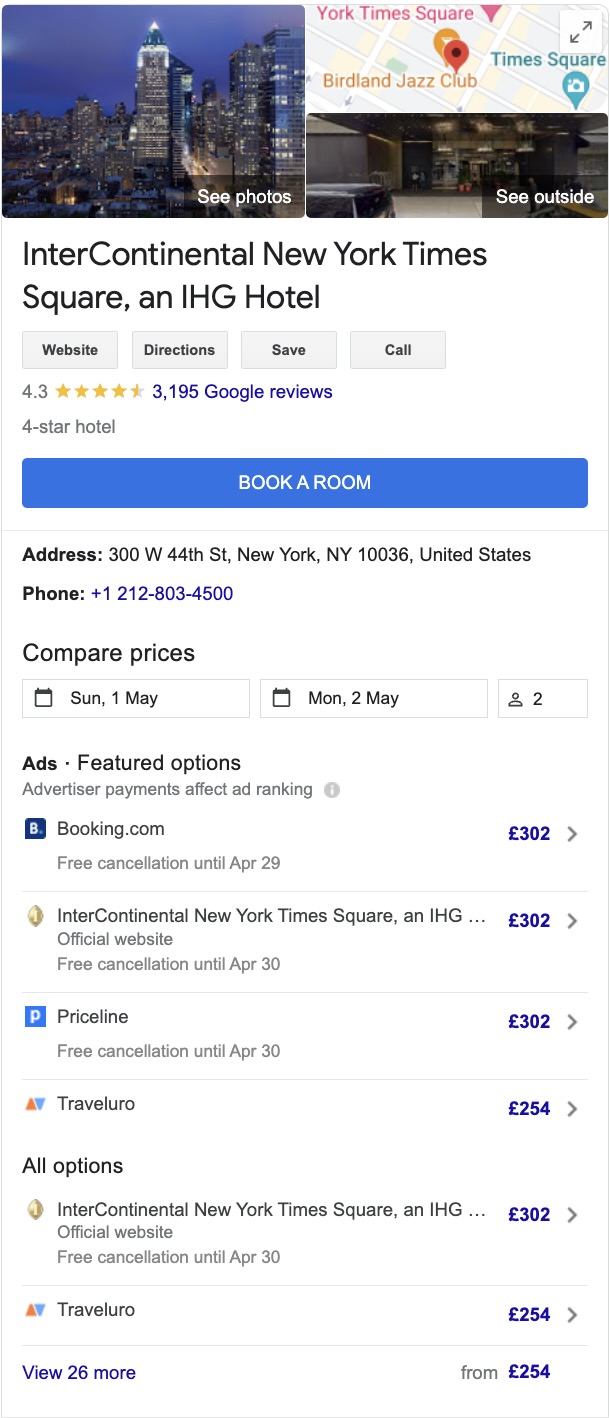The image appears to showcase options for booking a hotel room, specifically for the Intercontinental New York Times Square, an IHG Hotel. In the upper left corner, there is a photograph of high-rise buildings, suggesting a cityscape view. To the right, a prompt says "see photos," likely offering a gallery of the hotel and its surroundings. Additionally, there’s a map labeled "see outside" with another small photo below, enhancing the visual understanding of the hotel's location.

The hotel is identified as Intercontinental New York Times Square, an IHG Hotel, prominently displayed in the image. There are various interactive buttons, including "website," "directions," "save," and "call," providing users with different avenues for engagement. The hotel has a rating of 4.3 stars based on 3,195 Google reviews and is classified as a four-star hotel. 

A large blue button labeled "book a room" stands out on the page, urging immediate action. The hotel’s address is listed as 300 West 44th Street, New York, New York, followed by a phone number, which is highlighted in blue: 1-221-212-803-4500.

Below the booking button, there’s a section titled "compare prices" for a stay from Sunday, May 1st to Monday, May 2nd for two people. It shows various booking platforms and their offers:
- Booking.com: Offers free cancellation until April 29th for £302.
- Intercontinental New York Times Square (official website): Offers free cancellation until April 30th for £302.
- Baseline: Offers free cancellation until April 30th for £302.
- Traveluro: Offers a lower rate of £254.

An ad disclaimer notes that "featured options" may be influenced by advertiser payments affecting the ad rank.